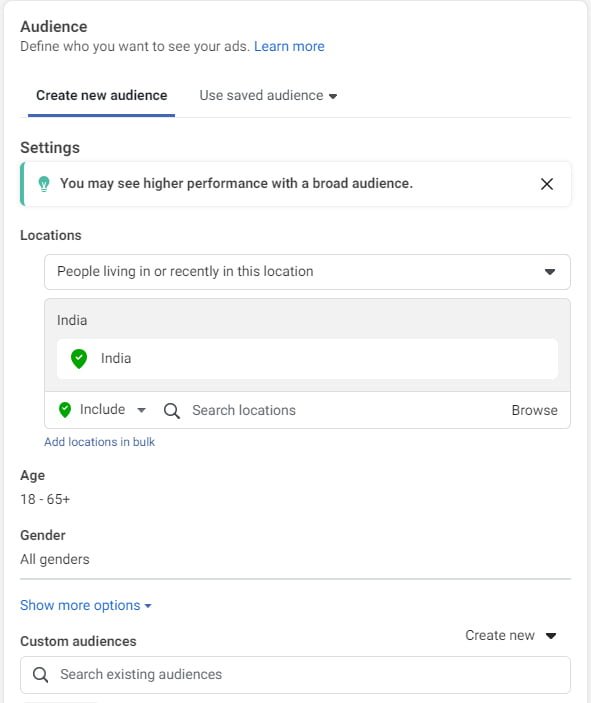Image Description: 

The image depicts a page with a white background, featuring various UI elements related to audience targeting for advertisements. 

In the upper left corner, the title "Audience" is prominently displayed in capital letters. Below this, in gray text, it says "Define who you want to see your ads," followed by a blue "Learn more" hyperlink. 

Moving down, there are two options: the first option, "Create New Audience," is highlighted in black text with a blue underline, indicating it is currently selected. The second option, "Use Saved Audience," is in gray text with a downward pointing arrow next to it.

Under these options, there is a section titled "Settings” in black capital letters. This is followed by an informational banner, which has a blue trim on the left side and a blue bulb icon. Within the banner, black text states, "You may see higher performance with a broad audience." There is a black 'X' on the right side of this banner to presumably close the notification.

Below the banner, the section titled "Locations" is in black text, followed by a white banner that reads "People living in or recently in this location" accompanied by a black downward arrow. Under this is a gray banner with the label "India" in the upper left corner. Within this gray banner is a smaller white banner featuring a green checkmark icon and the word "India."

Following this, there is another white banner containing a green checkmark icon, the word "Include," along with a downward arrow. Adjacent to this is a magnifying glass icon with the text "Search locations and browse." Beneath that, a blue hyperlink reads "Add locations in bulk."

Continuing down, the section labeled "Age" with a capital A specifies "18 to 65+." The next label says "Gender" and designates "All genders." A gray line divides this section, and beneath it, in blue text, are the words "Show more options."

The final section, "Custom Audiences," is noted in black text. To the far right of this section, it says "Create New" with a downward arrow. At the bottom of the image, there's a search bar with a magnifying glass icon and the placeholder text "Search existing audiences."